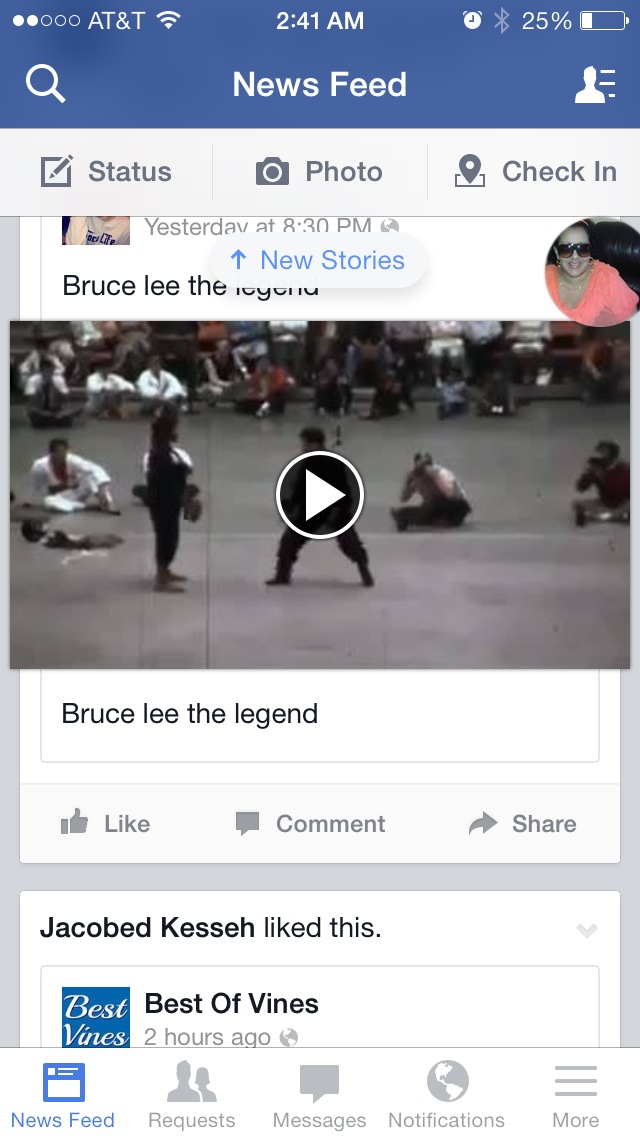The image is a detailed screenshot of a Facebook News Feed page displayed on a phone at 2:41 AM with 25% battery, showing an interface with blue and gray elements. At the very top, it says "News Feed" on the left, includes an hourglass symbol, and on the right, there's a silhouette of a person's head with three lines. Just below, on a white background, it lists options: "Status," "Photo," and "Check In."

Centrally, there's an oval circle labeled "News Stories" in blue text with an up arrow behind, noted as updated "Yesterday at 8:30 PM." Below this, the text "Blue Sleeve The Legend" appears, next to a circle featuring a woman's profile picture—she's wearing dark sunglasses and a pink shirt. The centerpiece of the screenshot is a video with a play button, depicting a group of people preparing for a karate tournament. Beneath the video, the caption repeats: "Blue Sleeve Legend."

At the bottom of the post, interaction options are listed in gray: "Like," "Comment," and "Share," followed by "Jacob Kinnish." Further down, it states "Best of Finds, Best of Finds 2 hours ago." At the very bottom, there are tabs for "News Feed," "Requests," "Messages," "Notifications," and "More." Additionally, a Messenger pop-up from a woman in a pink shirt is visible, indicating active social media engagement. The phone is noted to be using AT&T services.